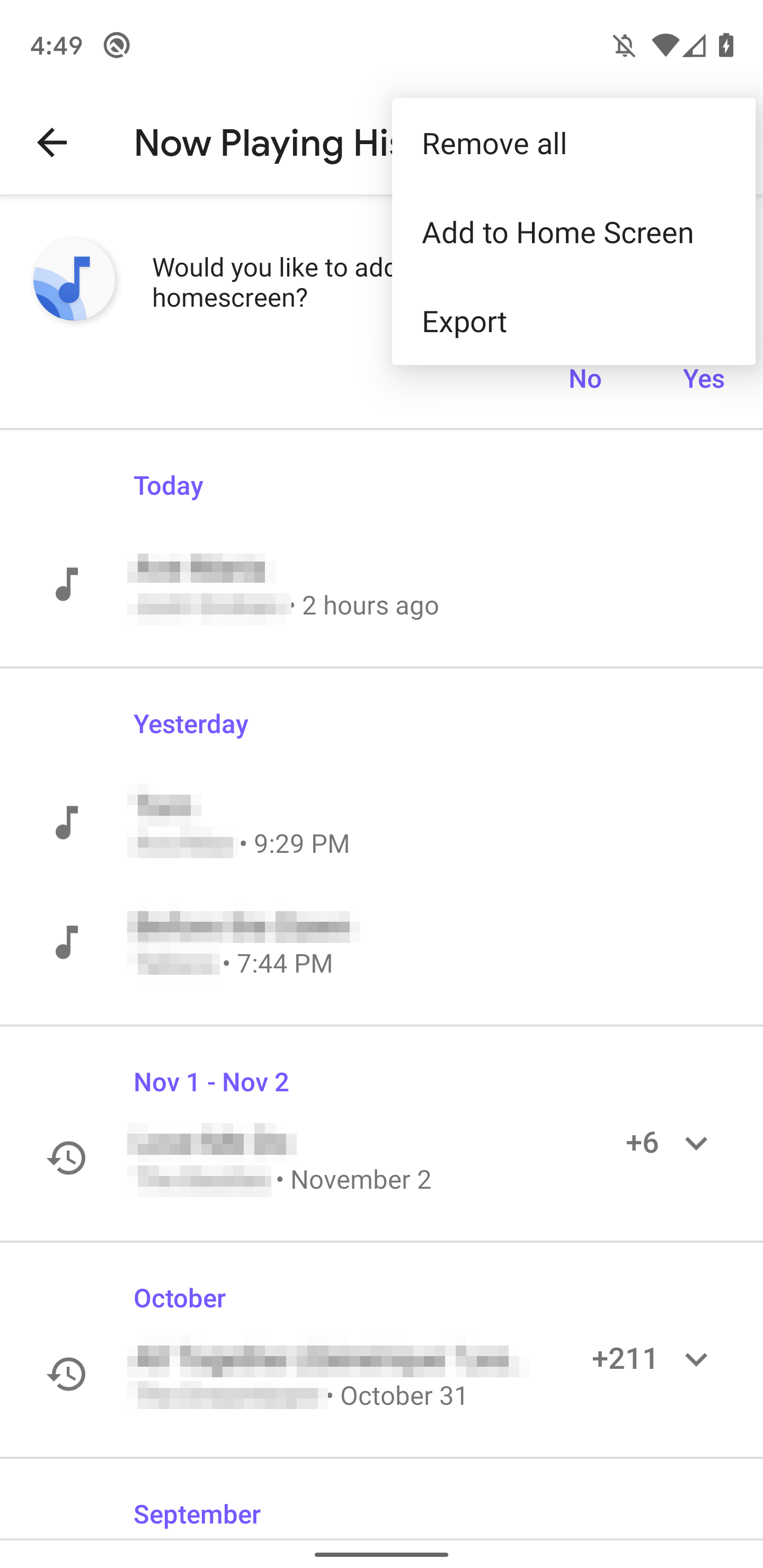A detailed screenshot captured from a cell phone screen. The image features a predominantly white background with some text in purple near the top. In the upper left corner, the time is displayed as 4:49, while the top right corner showcases a notification bell with a line through it, indicating silenced notifications. The Wi-Fi signal strength, network provider signal strength, and battery icon are also visible in the top right corner.

A white pop-up box occupies the top right quarter of the screen. This box contains three options: "Remove all," "Add to home screen," and "Export." Behind the pop-up box, an arrow pointing left is partially visible next to the blocked text that mentions "Now Playing" or something similar. Below this, there is a white circle with a blue music note icon inside, partially blue at the bottom left corner. Next to the icon, partially obscured by the pop-up box, the text starts with "Would you like to add" and continues with options "Home screen," "No," and "Yes."

Below, the screen is divided by a light grey line, beneath which the text "Today" appears next to a music note icon. The specific music details are blurred out. Following is another thin grey line leading to "Yesterday," coupled with two music notes, with the played content similarly blurred out. Another thin grey line precedes the date range "November 1st to November 2nd," featuring a time symbol and the text "plus 6" with a drop-down arrow; the music details are still blurred out. The line below marks "October" in purple, next to a clock symbol, displaying "211" entries with a drop-down arrow. Just visible at the bottom is the beginning of the word "September."